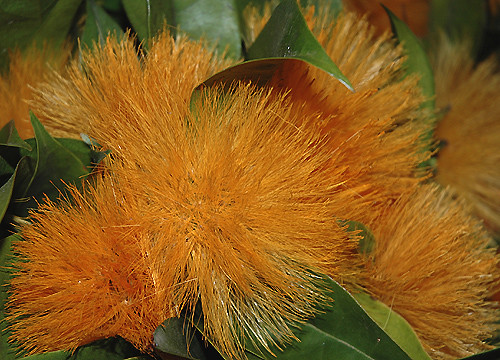This digital photograph showcases a close-up of a vibrant plant, featuring striking burnt orange, fluffy spherical flowers that resemble the fluff on a toboggan hat. There are approximately four or five of these intricate, golf ball-sized orbs, each with a furry texture, giving the plant a whimsical appearance. The lush, bright green leaves, numbering around ten to fifteen, contrast vividly with the orange buds and appear partially obscured by them, contributing to the dense and intriguing composition of the image. One leaf is particularly noticeable as it pokes through the floral elements, further emphasizing the lush and healthy nature of the plant. The photograph's close-up perspective intensely highlights the interplay of colors and textures, offering a detailed and mesmerizing view dominated by these unique spherical blooms and verdant foliage.